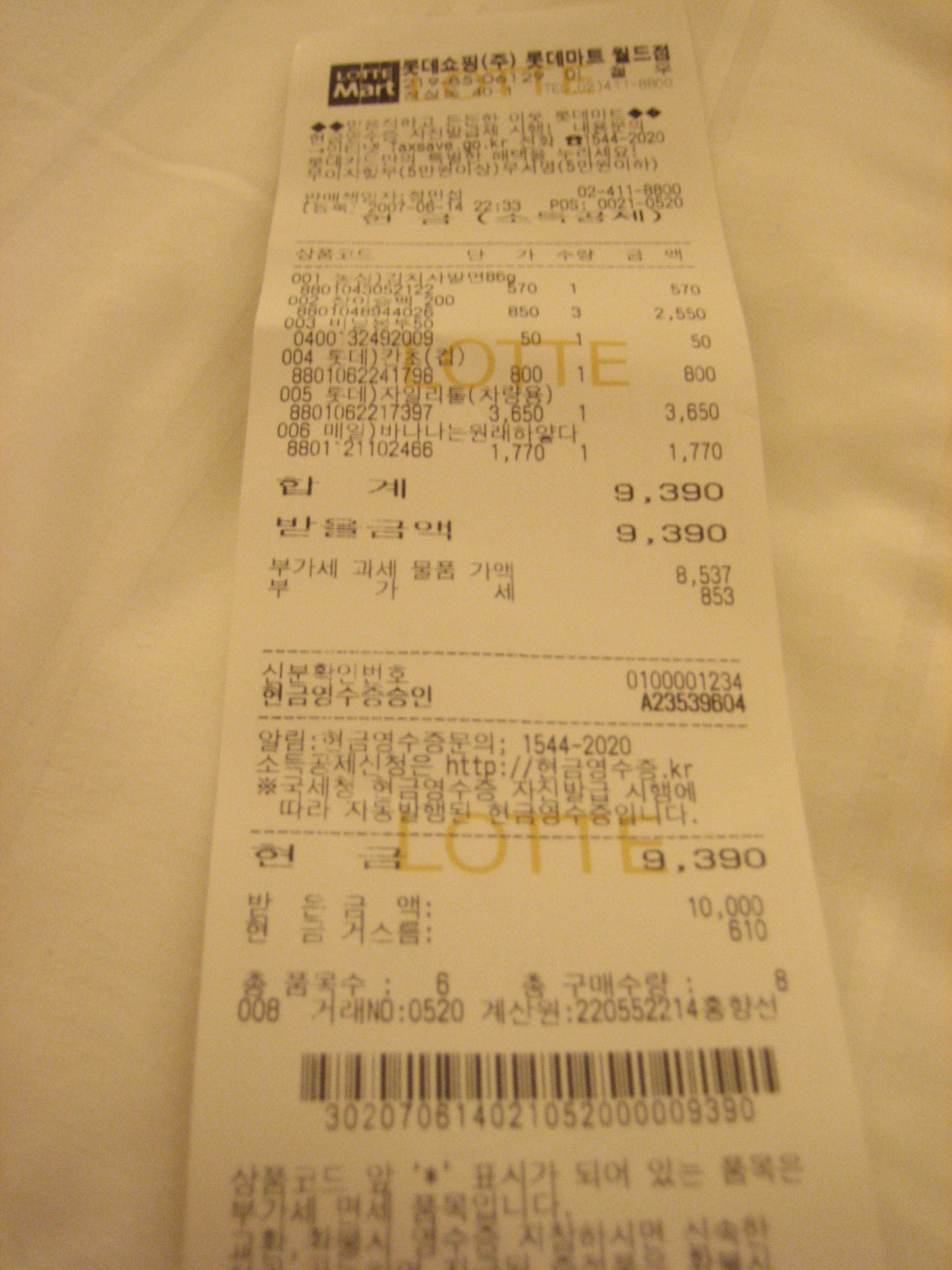The image shows a photograph of an actual registered receipt, written in an unidentified Asian language. The receipt is laid out on a piece of fabric, possibly a tablecloth or blanket. At the top, the name of the business is prominently displayed in the foreign script, accompanied by a few numbers. Below this, the receipt details various items purchased, each identified by a unique 10-digit UPC number on the left, with corresponding prices aligned on the far right. The total amount of the purchase is highlighted in bold, and the payment method is indicated. Further down, the transaction continues, culminating in a 16-digit receipt ID number. Additional text in the foreign language appears at the bottom of the receipt.